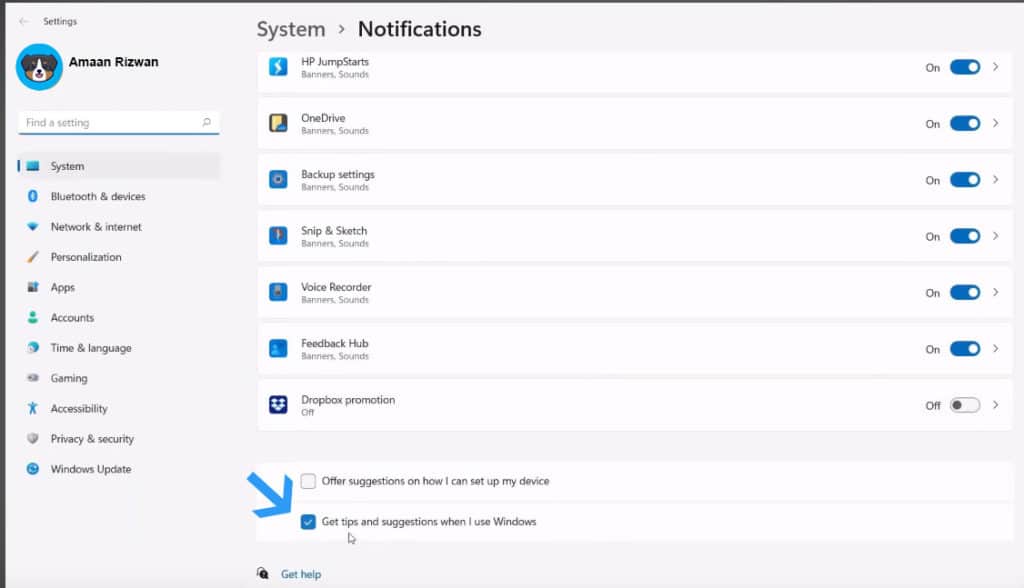The image is a screenshot of a computer's settings interface. In the upper left corner, the word "Settings" is prominently displayed, while to its right, "System Notifications" can be seen. Below "Settings," there is a blue square containing a picture of a dog and the name "Amin Rizwan." Directly beneath that, a search bar labeled "Find a setting" is visible.

On the left side of the screenshot, a vertical list of categories is displayed, including: 
- System
- Bluetooth and Devices
- Network and Internet
- Personalization
- Apps
- Accounts
- Time and Language
- Gaming
- Accessibility
- Privacy and Security
- Windows Update

To the right side of the image, multiple settings are being managed. The following are toggled on:
- HP Jump Start
- OneDrive
- Backup settings
- Snip & Sketch
- Voice Recorder
- Feedback Hub

Additionally, "Dropbox Promotion" is toggled off. At the bottom of this section, there are two options:
1. "Offer suggestions on how I can set up my device"
2. "Get tips and suggestions when I use Windows" (which has a check mark next to it and a blue arrow pointing towards it).

The overall screenshot provides a detailed view of various settings and configurations available on the computer, highlighting the current state of system notifications and other preferences.